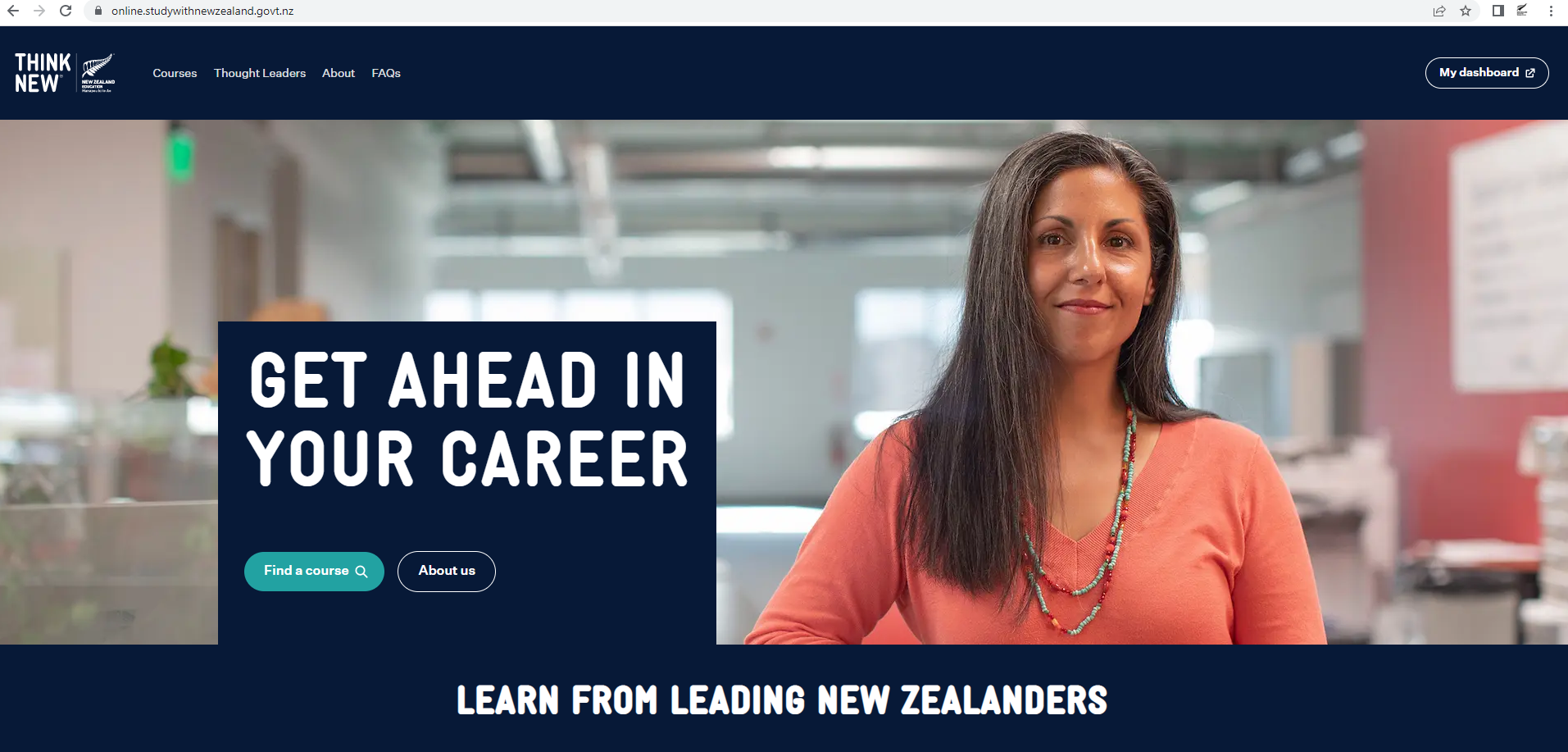This webpage offers resources for advancing your career, featuring tools to find various courses. It includes tabs such as "About Us" and "Frequently Asked Questions," suggesting the importance of user guidance and transparency. The website appears to be New Zealand-based, highlighting learning from leading New Zealand professionals. The design includes a navy blue header and footer for a cohesive look. Centrally, there's an image of a large office space with a woman seated to the right. She has long dark hair, is dressed in an orange top and beaded necklaces, and is smiling warmly at the camera.